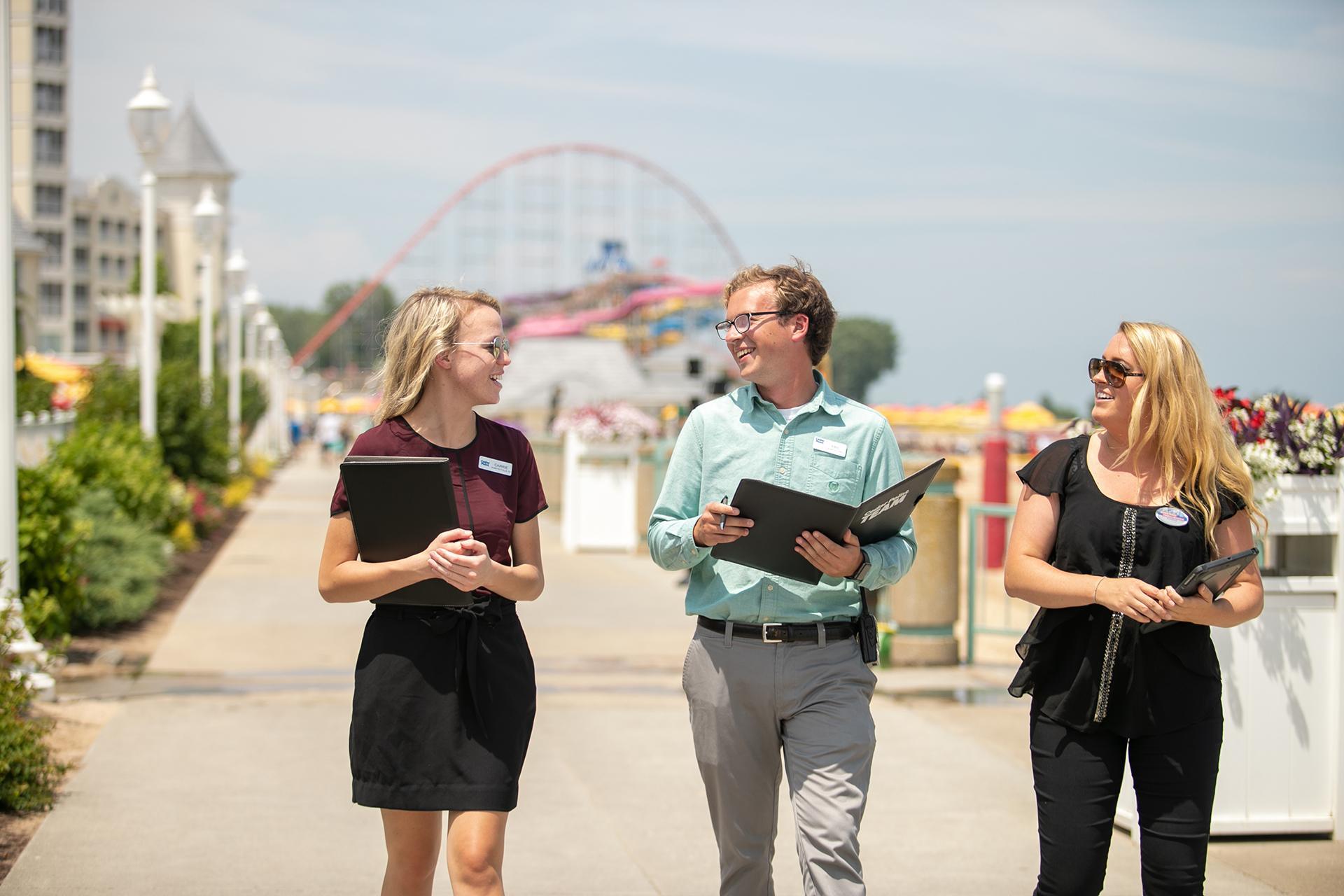The image depicts a lively scene on a sunny boardwalk, distinguished by a clear, light blue sky. In the distant background, a vibrant red roller coaster and various amusement park rides, along with some tall white buildings with numerous windows, create an exciting atmosphere. The boardwalk is flanked by a line of white lampposts and lush shrubbery, adding to the scenic ambiance. 

Prominently in the foreground, three people engage in a cheerful conversation. To the left stands a woman with long blonde hair, wearing a short-sleeved maroon top and a black skirt that reaches just above her knee. She carries a book or folder and wears glasses, as well as a name tag on the top right of her outfit. 

The man in the middle, sporting glasses, has dark short hair and dons a long-sleeved light green shirt paired with grey pants and a black belt. He also holds a black folder or book and has a pen in his hand, with a similar name tag attached to his shirt. 

To the right is another woman with long blonde hair. She is adorned in a black short-sleeved top and black pants. Like the others, she holds a booklet close and has glasses and a name tag, albeit hers is oval-shaped, positioned at the top right of her attire. Together, this trio’s relaxed demeanor and engaged interaction capture the joyous spirit of a bright day at what seems to be a bustling amusement park or resort boardwalk.